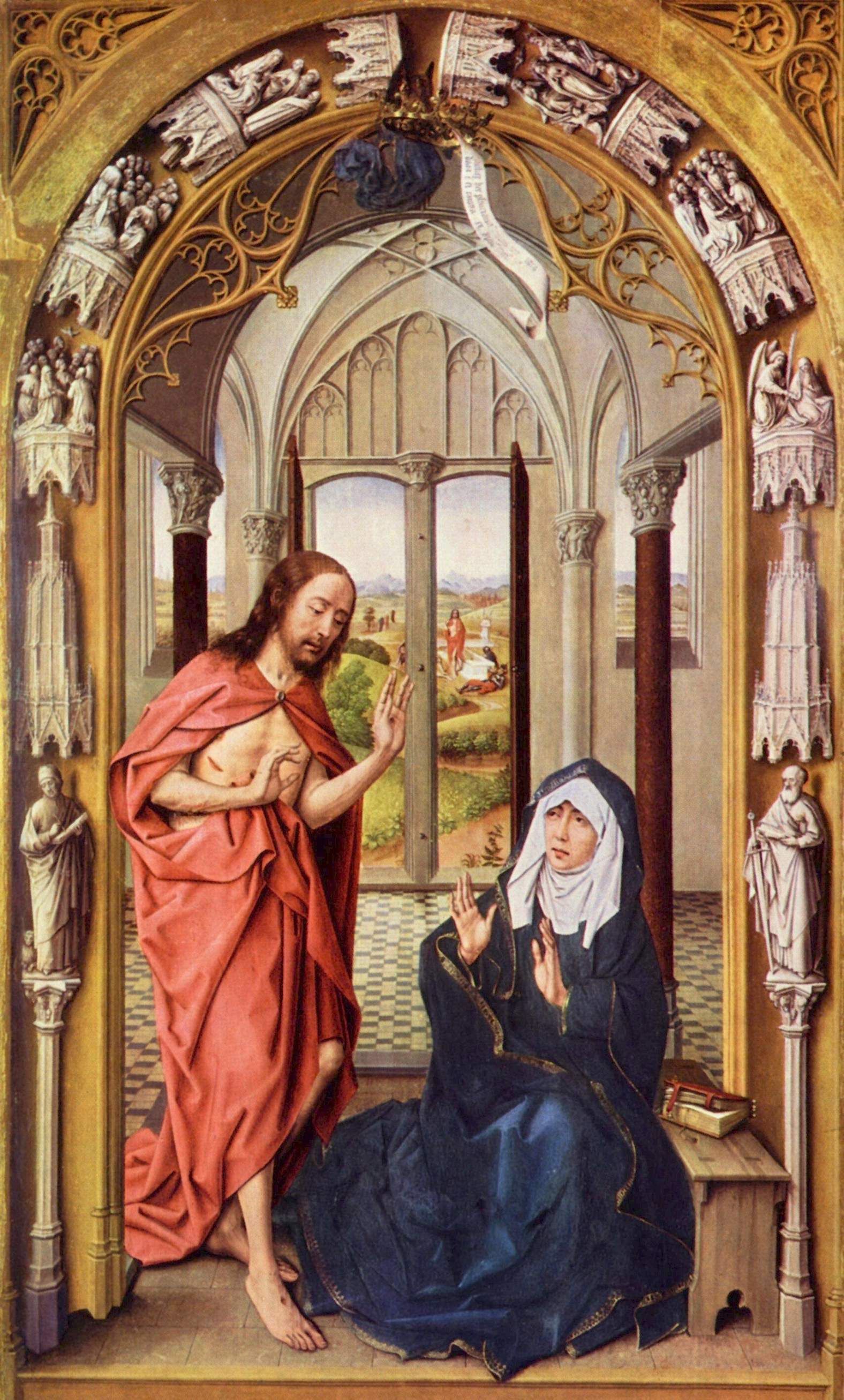The image depicts a detailed religious art piece set beneath a richly adorned archway. At the center stands Jesus, clearly identifiable by the wounds on his hands, feet, and side, dressed in an orangey-red robe. His physical appearance includes long, reddish-brown hair, a thin build, and a shadow of a beard. He stands in a doorway which appears to be part of an ornate church, with domed structures and intricate carvings surrounding the archway. These carvings feature an array of figures including men holding tablets and scepters, angels, and crowned sculptures, possibly rendered in marble. 

In front of Jesus, kneeling, is a woman who presents as Mary Magdalene or possibly a nun. She is dressed in a dark, full dress with a head covering, consisting of a black veil over a white habit. Her expression is one of astonishment as she gazes up at Jesus, suggesting she has just witnessed his resurrection.

The interior of the setting includes marble columns and a patterned tile floor. Behind the woman, there is a wooden bench with an open book, indicating she might have been studying before this miraculous event. The background of the scene includes a window that reveals a pastoral landscape with rolling green hills and distant figures, enhancing the serene and holy atmosphere of the artwork.